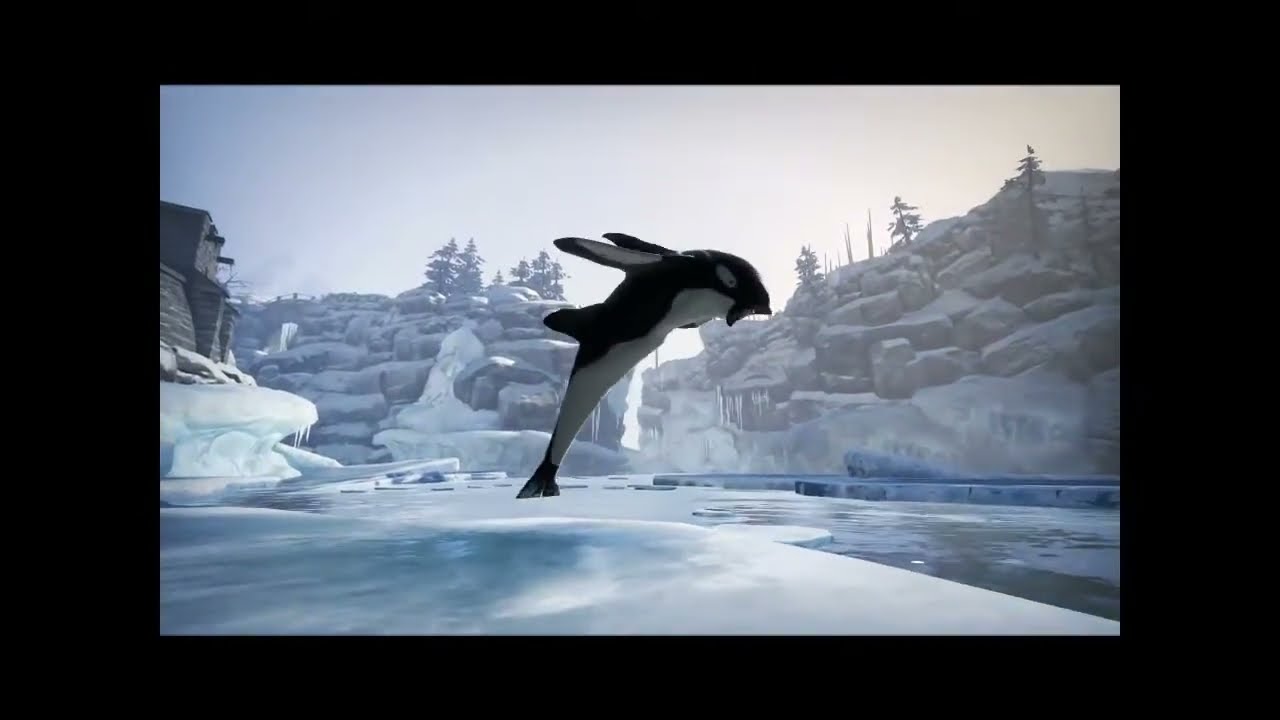In this AI-generated image, framed with a thick black border on the sides and a thinner top and bottom, a surreal winter Arctic scene unfolds. Snow-capped mountains with scattered pine trees dominate the background, while a stone building perched on a rocky, icy ledge is visible on the right. The foreground features a mix of snow and an icy river or sepia-toned water, radiating light. The focal point is a fantastical creature—a cross between an orca whale and a seagull—leaping majestically out of the water. The creature's body resembles an orca with a curved tail and dorsal fin, but it has seagull-like wings sprouting from its back. Adding to its whimsical appearance, the creature also sports black rabbit ears and a mustache. The sky above is a muted gray, enhancing the ethereal, otherworldly atmosphere of this striking image.